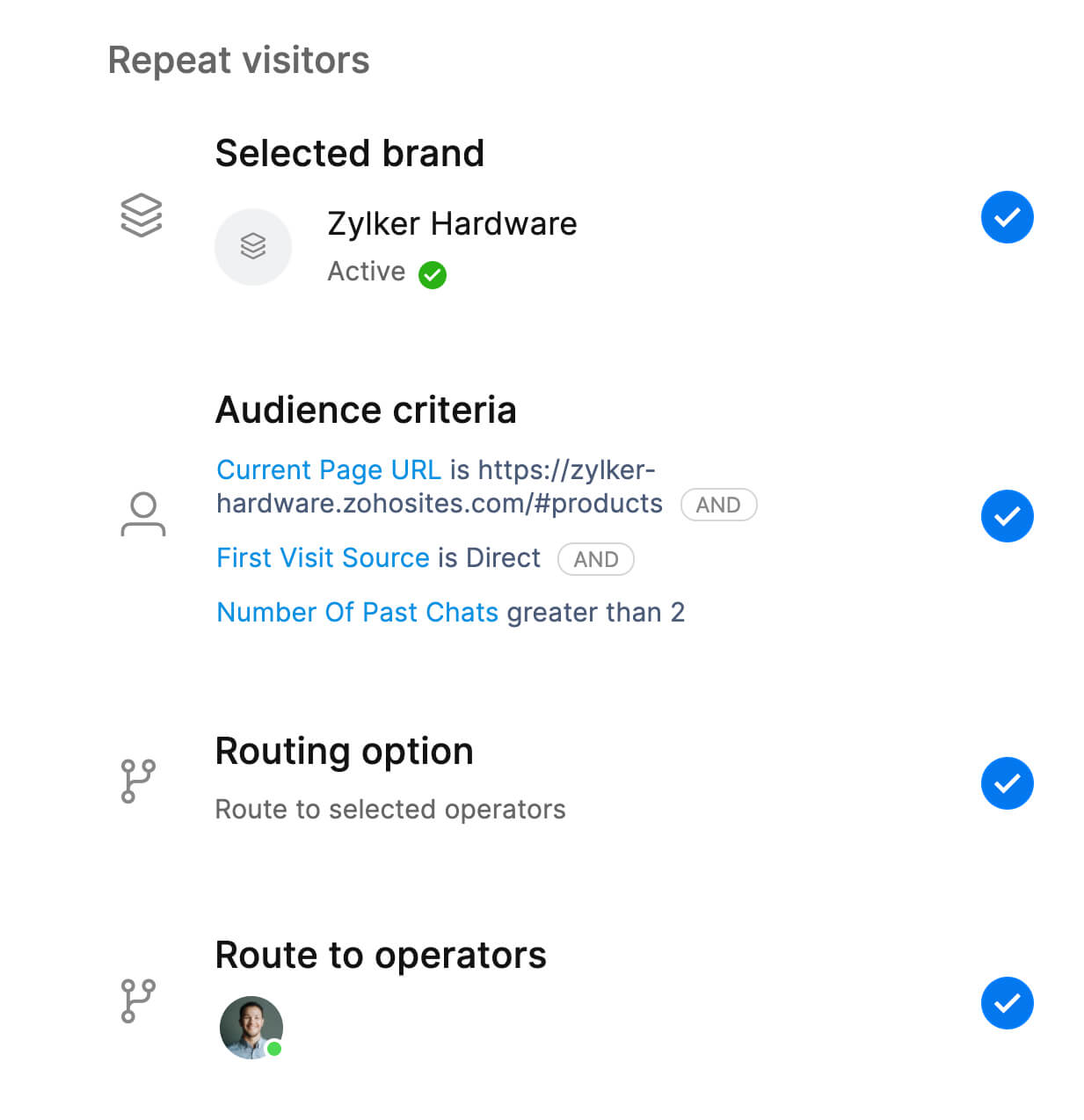Screenshot Caption: 

The screenshot showcases a section titled "Repeat Visitors," featuring specific visitor metrics and routing options. 

1. **Selected Brand**:
   - Icon: Three stacked squares
   - Brand: ZYLKER Hardware
   - Status: Active (indicated by a green circle with a checkmark)
   - Additional Indicator: Blue circle with a white checkmark

2. **Audience Criteria**:
   - Icon: Person
   - Categories underneath:
     - **Current Page URL**: zykerhardware.zoho.sites.com, etc.
     - **First Site Source**: Direct, etc.
     - **Number of Past Chats**: Greater than two
   - Indicator: Blue circle with a white checkmark

3. **Routing Option**:
   - Icon: Three interconnected circles
   - Description: Route to selected operators
   - Indicator: Blue circle with a white checkmark

4. **Routing to Operators**:
   - Icon: Three interconnected circles
   - Description: Route to operators
   - Operator's Profile: 
     - Picture: White male with dark hair, smiling, wearing a dress shirt
     - Status: Active (indicated by a green circle in the bottom right of the picture)
     - Additional Indicator: Blue circle with a white checkmark

Each section and detail meticulously provides insight into the categorization and routing setup for repeat visitors to ZYLKER Hardware’s online presence.